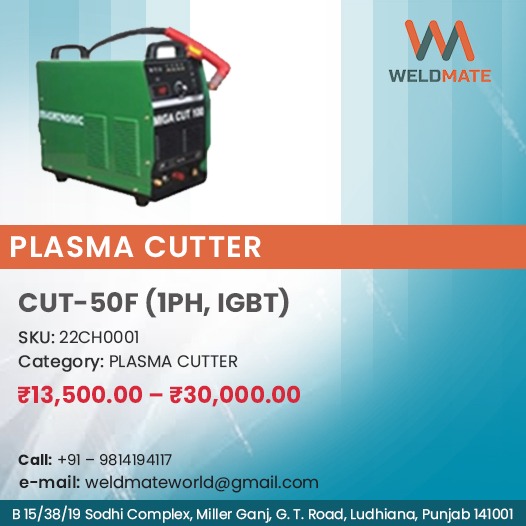The advertisement image is for a plasma cutter by Weld Mate, featuring a blue background with varying shades of blue lines. In the top left corner is an image of the plasma cutter, which has green sides and white writing, with the front end displaying different colored knobs and buttons (red, yellow, white). It also has a red, gun-like attachment. The machine prominently features the words "Mega Cut" on the front. 

On the top right, the Weld Mate logo is displayed with a distinctive W and M combined in a wavy black and red design, followed by the words "weld" in black and "mate" in red. Below this, the model is identified as "Plasma Cutter CUT-50F," with additional details in parentheses indicating "1PH, 1GBT." The SKU number, product category (plasma cutter), and price range ($13,500 to $30,000) are listed.

The advertisement concludes with a call number, email address (weldmateworld@gmail.com), and a physical address at B-1538, 19 Soty Complex, Miller Gange, GT Road, Ludhiana, Punjab, 141001.